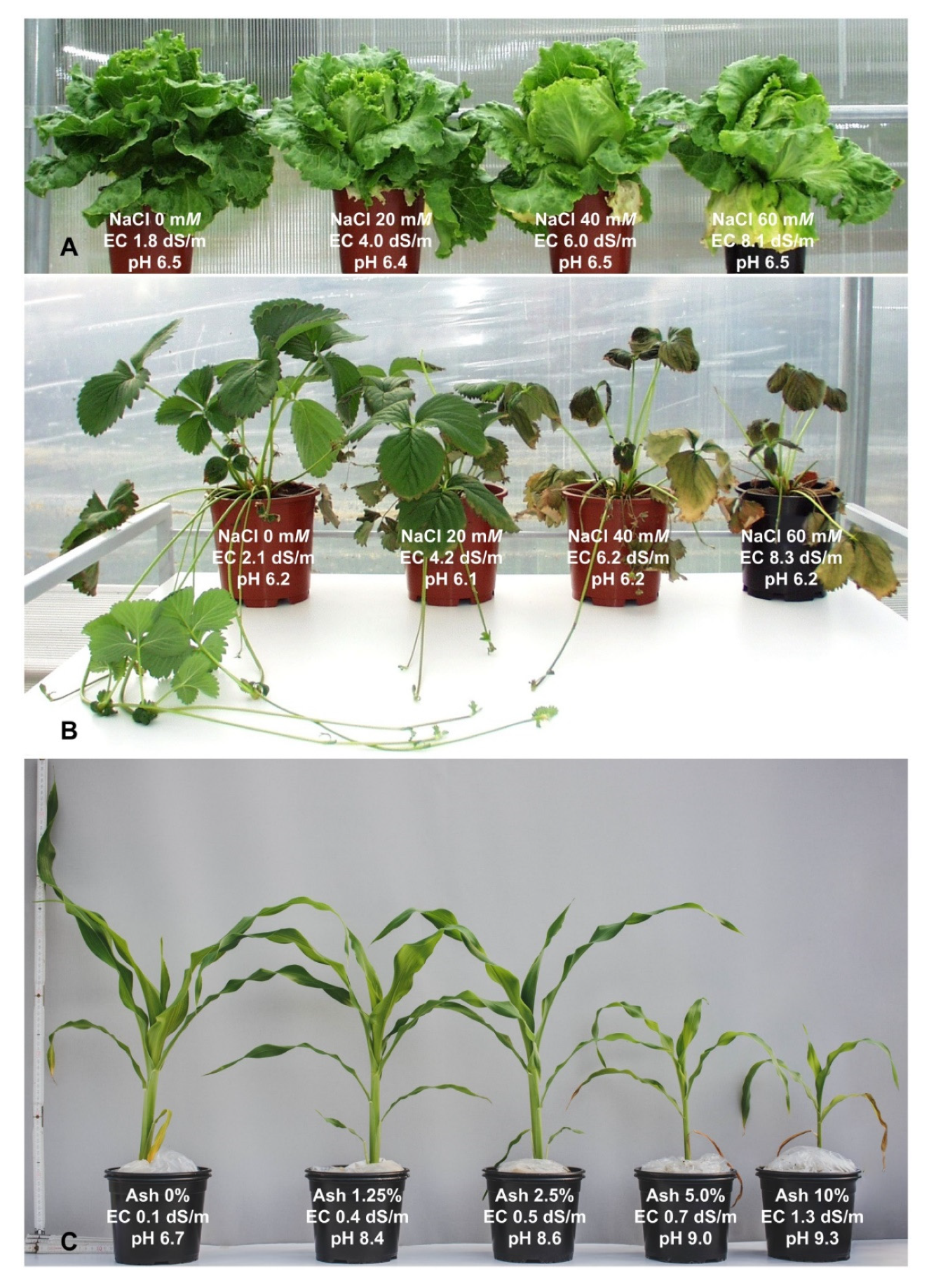The image is divided into three distinct segments of varying sizes, each labeled with black letters on a gray background. The top segment (A) showcases four pots containing full-grown heads of lettuce, positioned against a gray backdrop. Each pot is marked with white, scientific, or chemical notations, which include varying pH levels such as 6.5 and 6.4. The middle section (B) features four vine-style houseplants in red pots, sitting on a white table. These plants also bear white scientific labels indicating different treatments or conditions. The bottom segment (C) displays five pots with tall corn stalks emerging from them, set on a light-gray table against a white background. This section also includes white-lettered labels on the pots, such as ash content percentages and pH levels, indicating a scientific study on the effects of different treatments on plant health and growth. The overall visual illustrates comparative growth studies, showing how different conditions affect each set of plants, with controls usually appearing healthier and more vigorous than the treated ones.